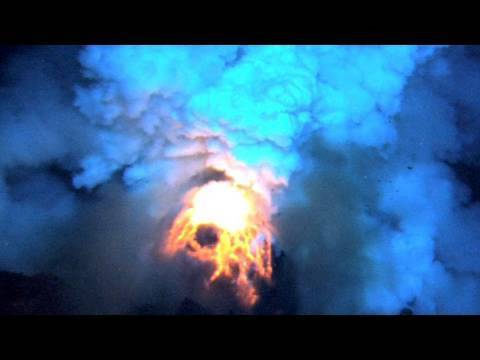The image captures the dramatic eruption of an undersea volcano, showcasing a striking contrast of colors and elements. Plumes of bluish-white smoke and dust billow out from the volcanic site, blending with the surrounding blue water. The central focus is on the vivid red and yellow lava, spurring out and creating a mesmerizing, fiery spectacle against the cooler tones of the ocean. The image appears to be taken from an Odin-type camera or drone footage, evident from the aerial perspective and the letterboxed black bars across the top and bottom, hinting at a screenshot from a video. The scene is illuminated by the bright, intense glow of the erupting magma, emphasizing the raw power and beauty of this natural event.